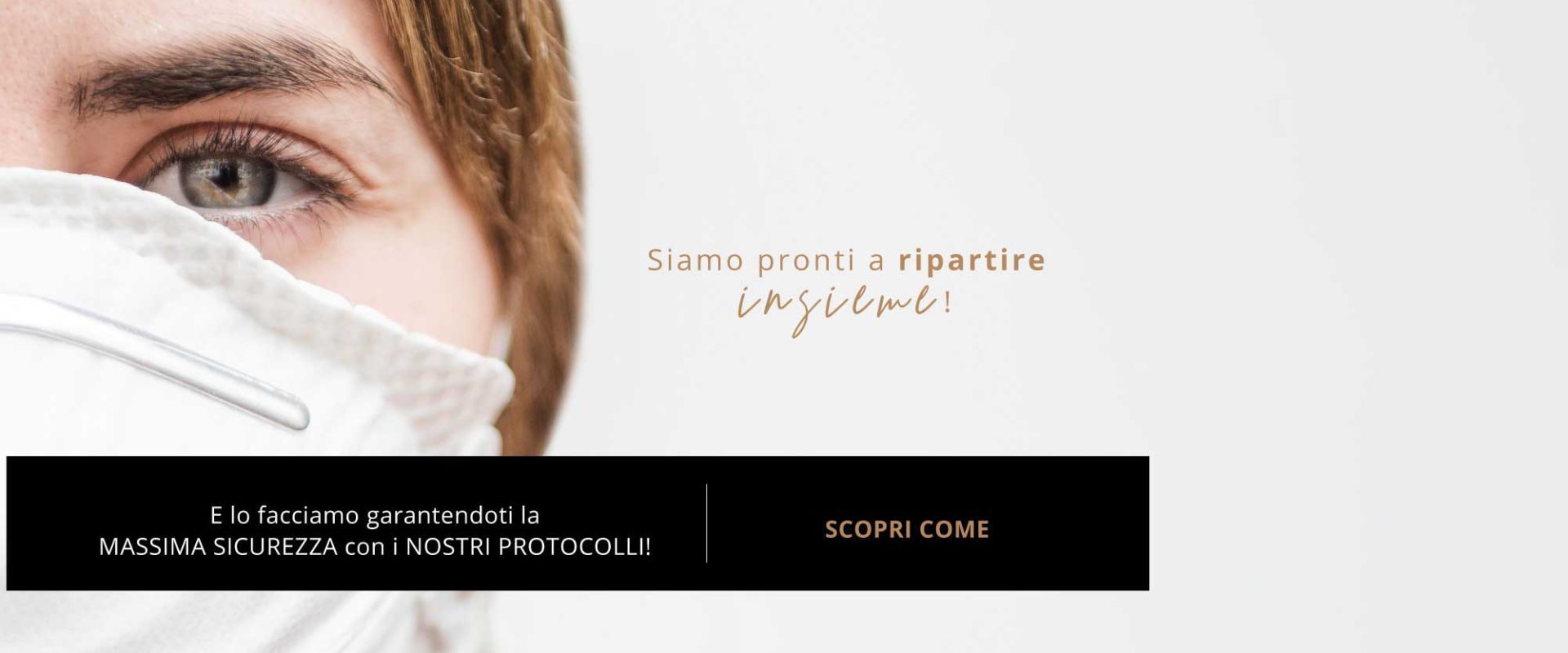The image displays the right side of a person's face, most likely a woman, wearing a white cloth face mask. Only the area from the nose to just above the eyebrow is visible. The person has meticulously groomed, dark eyebrows, gray eyes, and reddish or strawberry blonde hair. The background is white. 

Adjacent to the face is an Italian advertisement, partially legible, with some text in a golden, cursive font and other parts in white within a black rectangular block. The text includes: "Siamo Pronti a Ripartire" and "E lo facciamo garantendoti la massima sicurezza con i nostri protocolli." There is also a vertical gold line separating another piece of text that reads, "Scopri come."